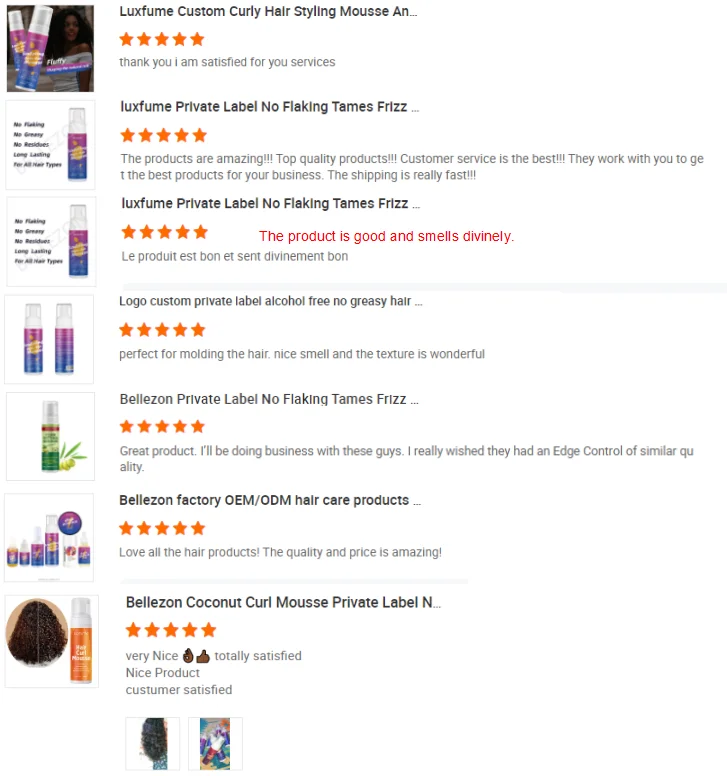Luxfume Curly Hair Styling Mousse: A satisfied customer's review highlights the exceptional quality and effectiveness of the Luxfume custom curly hair styling mousse. The mousse, which comes with a private label and logo customization, is praised for being alcohol-free and not leaving any greasy residue. It effectively tames frizz without causing flaking and has a divine fragrance. The customer emphasizes their complete satisfaction with the product and the stellar customer service. Additionally, the Belazon Coconut Curl Mousse is mentioned favorably for its similarly high quality in private label hair care products offered by the Belazon factory, which specializes in OEM/ODM services. The reviewer expresses their love for both brands' hair care products and appreciates their competitive pricing and overall quality. They express a desire for an edge control product of comparable quality.